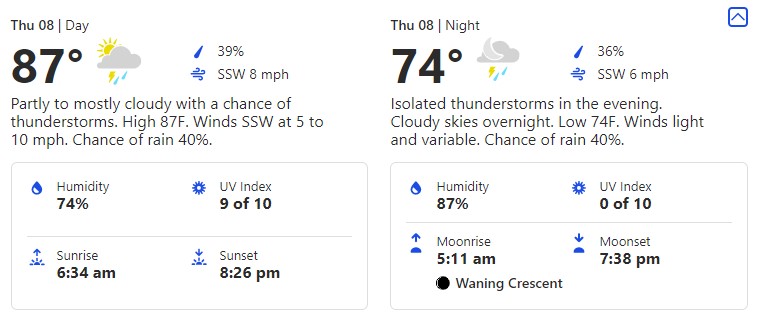The image is a horizontally oriented weather forecast display that is approximately two and a half to three times wider than it is tall. The background is entirely white, which creates the appearance of no definite perimeter. The display is symmetrically divided into two equal halves, resembling two windows showing data for different times of the day—daytime on the left and nighttime on the right.

In the upper left corner of both sections, the date is clearly marked as "Thursday the 8th," abbreviated to "THU 08." Each half is labeled respectively with "Day" on the left and "Night" on the right, separated by a vertical line. 

The daytime section details an 87-degree temperature in bold black text, accompanied by an icon showing a rain cloud with a sun partially obscured behind it, a lightning bolt beneath, and raindrops. To the right of the cloud icon, it indicates a 39% chance of rain with a small raindrop icon.

The nighttime section shows a somewhat lower temperature of 74 degrees, illustrated by a rain cloud with a moon behind it, lightning, and raindrops, similar to the daytime icon. Here, the chance of rain is slightly lower at 36%, denoted by an adjacent raindrop icon.

Below each weather depiction, there is an icon representing wind speed, visualized by three horizontal, blue candy cane-like lines pointing to the right. The daytime wind is noted as coming from the southwest at 8 miles per hour, while the nighttime wind is from the south-southwest at 6 miles per hour.